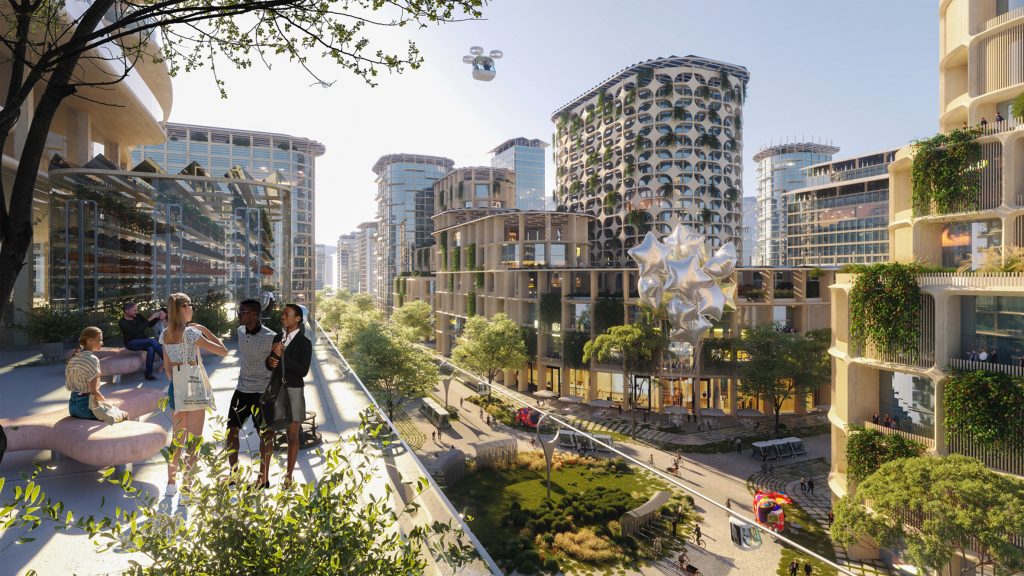In this captivating cityscape, a remarkable blend of futuristic and rural elements comes to life. Tall skyscrapers dominate the skyline, their reflective silver façades gleaming under the sun, while others are adorned with cascading green plants, intertwining nature with urban architecture. Forested areas flourish along the streets, providing a contrast to the towering buildings. A sizable drone, large enough to potentially accommodate a human, hovers near the top of the image, epitomizing the advanced technology integrated into everyday life. On the left, a small group of people—one woman and two men—engage in conversation, while several others relax on pale pink, leather-like benches. This unique cityscape, with its harmonious fusion of verdant greenery and cutting-edge infrastructure, offers a striking vision of coexistence between nature and modernity.